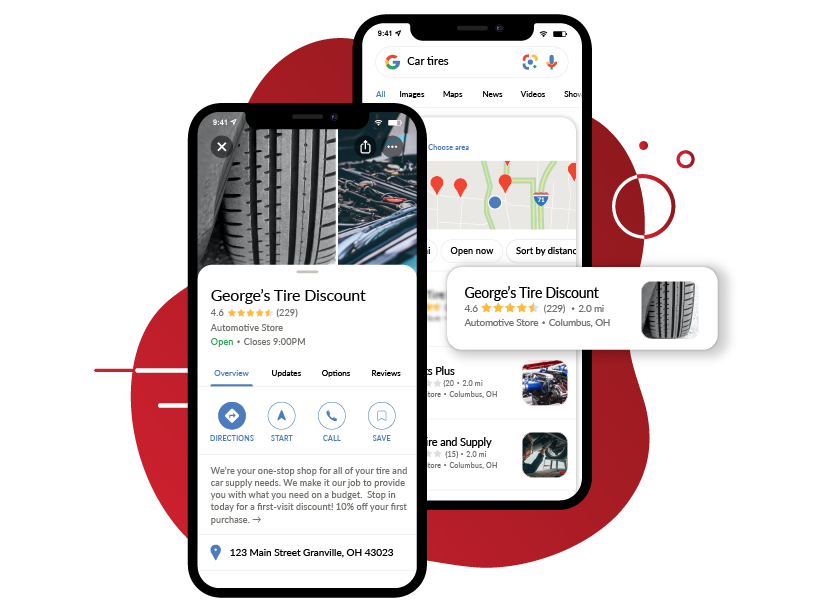The image features two smartphones placed on a white background, with a prominent red blob in the center of the backdrop. The red blob is distinctive, showing small bubbles emanating from its right side.

The smartphone on the left is framed with a black border. Its screen displays the top part of a black tire, emphasizing the tread detail. Below the tire image, the screen showcases a service titled "Georgia's Tire Discount," which has received a rating of 4.6 stars, indicated by star icons. The interface includes tabs labeled "Overview," "Updates," "Options," and "Reviews," with the "Overview" tab currently selected. Additionally, it appears that the user has opted for navigation directions. The screen also features a descriptive promotional message: "We're your one-stop shop for all your tire and car supply needs. We make it our job to provide you with what you need on a budget. Stop in today for a first night, first visit discount: 10% off your first purchase." The business location is specified as 123 Main Street, Granville, Ohio 43023.

Behind the first phone, the second smartphone screen appears to display search results for "Georgia's Tire Discount," offering various car tire options.